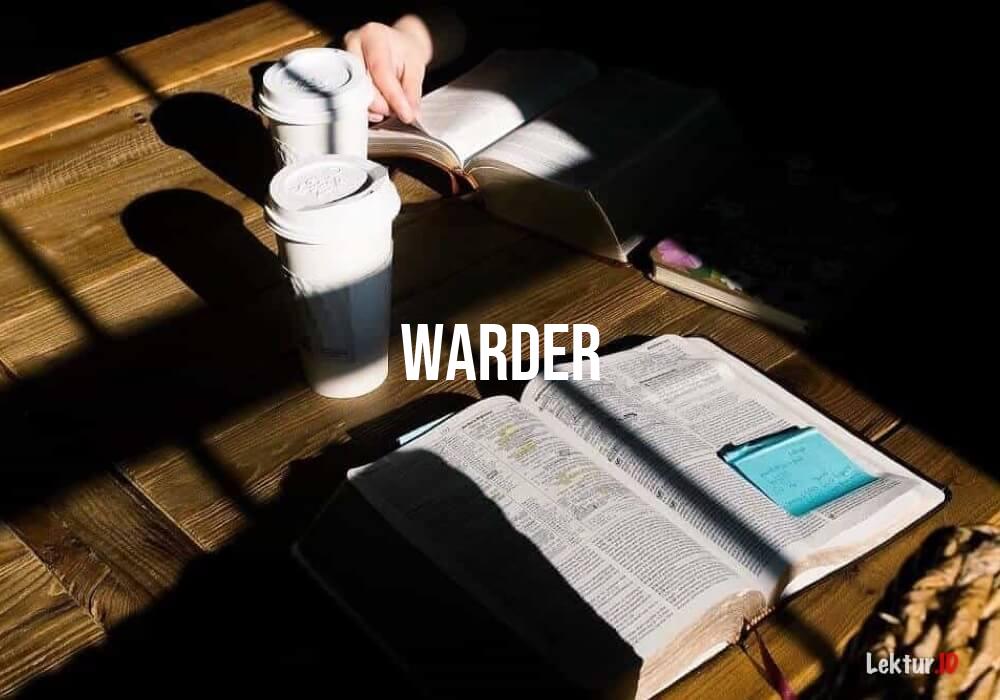The photograph captures an intimate scene at a rustic, dark wooden table in what seems to be a coffee shop, illuminated by sunlight that creates deep, almost pure black shadows. Two people are seated at 90 degrees from each other, each engrossed in a book. From the near perspective, we view an open book at a slight angle, as if we were reading it ourselves. This book, possibly a Bible, features pages adorned with blue sticky notes and gold-foiled edges, suggesting a sacred or important text. The other book is positioned catty-corner on the right, where a white hand is seen turning a page. Between the books, two white coffee cups with lids are placed centrally, accentuating the cozy, conversational atmosphere. The rich wood grain of the table runs diagonally from the left, contributing to the rustic charm. Adding a mysterious touch, white text reading "WARDER" appears prominently in the center of the image.